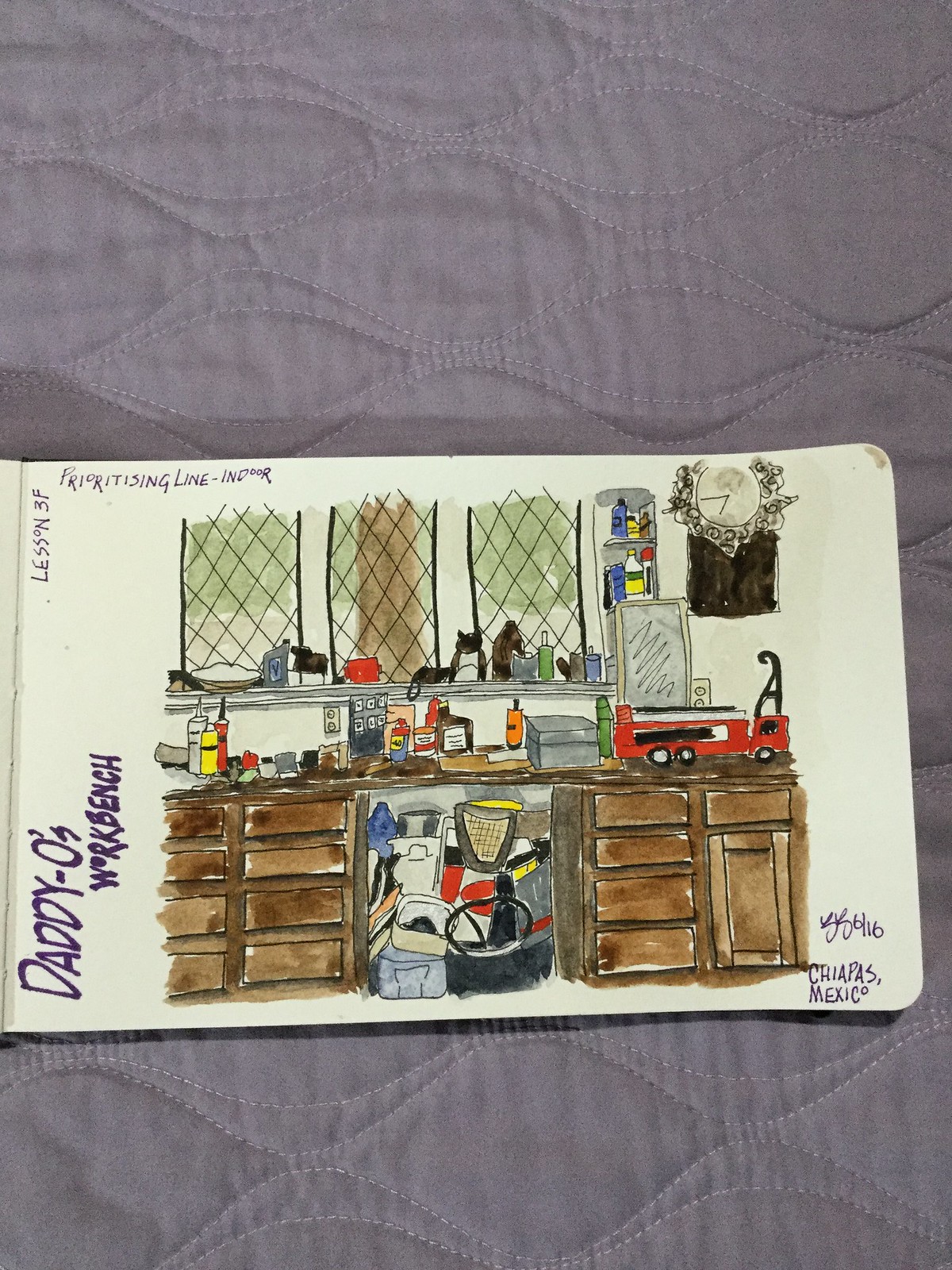The photo captures a detailed scene situated on a soft, purple bedspread, characterized by a circular weave pattern, possibly indicative of a blanket or mattress. Placed prominently on this textured background is an image resembling a postcard, featuring a chaotic workbench or kitchen setup.

The postcard's stark white background contrasts sharply with the cluttered and busy interior scene. Central to the image is a workbench laden with assorted tools and materials, seemingly epitomizing organized chaos. Various spray bottles and lubricants, including a recognizable WD-40 can, clutter the surface. Several drills and other tools are scattered across the bench, some even balanced precariously on the window and shelves near the workspace.

The backdrop of the workbench reveals barred windows through which a tree can be seen, infusing a hint of the outside world into this cramped, industrious setting. Adjacent to the windows, a small shelf adds to the clutter with more items perched haphazardly.

The workbench itself is robust and brown, featuring numerous closed drawers that conceal their contents, leaving their mysteries to the imagination. The upper right corner of the image showcases a miniature fire truck, providing a whimsical touch to the otherwise utilitarian scene. Above the workbench, a grandfather clock adorns the wall, adding a sense of timelessness to the photograph.

Below the workbench, the undercarriage between two potential seating spaces is packed with various items, likely stored for utility. The indistinct jumble of bags, tubs, and perhaps other miscellaneous gear suggests a makeshift storage solution, contributing to the overall impression of a busy and functional, albeit untidy, workspace.